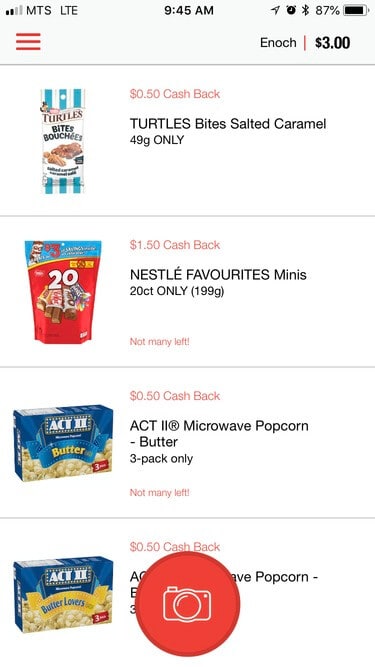The screenshot depicts an app interface of a cashback website focused on food purchases. At the top, the status bar displays details typical of a smartphone interface: the cellular LTE signal with two bars on the left, the time centered at 9:45 AM, and icons for Bluetooth, alarm, location services, and an 87% battery level on the right. 

Below the status bar, a red hamburger icon appears on the top left against a gray background. To the right, the text "Enoch" is prominently displayed in bold, alongside a red pipe symbol and "$3.00". 

The main section of the interface showcases four available products eligible for cashback, each accompanied by an image and cashback details in red text. The first product listed is "Turtle's Bite salted caramel, 49 grams," offering $0.50 cashback. The second product, "Nestle Favorites Mini, 20 count," provides $1.50 cashback and includes a note in smaller red text indicating "not many left." The final two products are examples of popcorn, each offering $0.50 cashback: "Microwave Popcorn Butter, three pack only." 

At the bottom of the screen, there is a dark red circle with a slightly smaller, lighter red circle inside, featuring a white camera icon. This button is intended for users to press to submit a picture of a receipt to claim their cashback rewards.